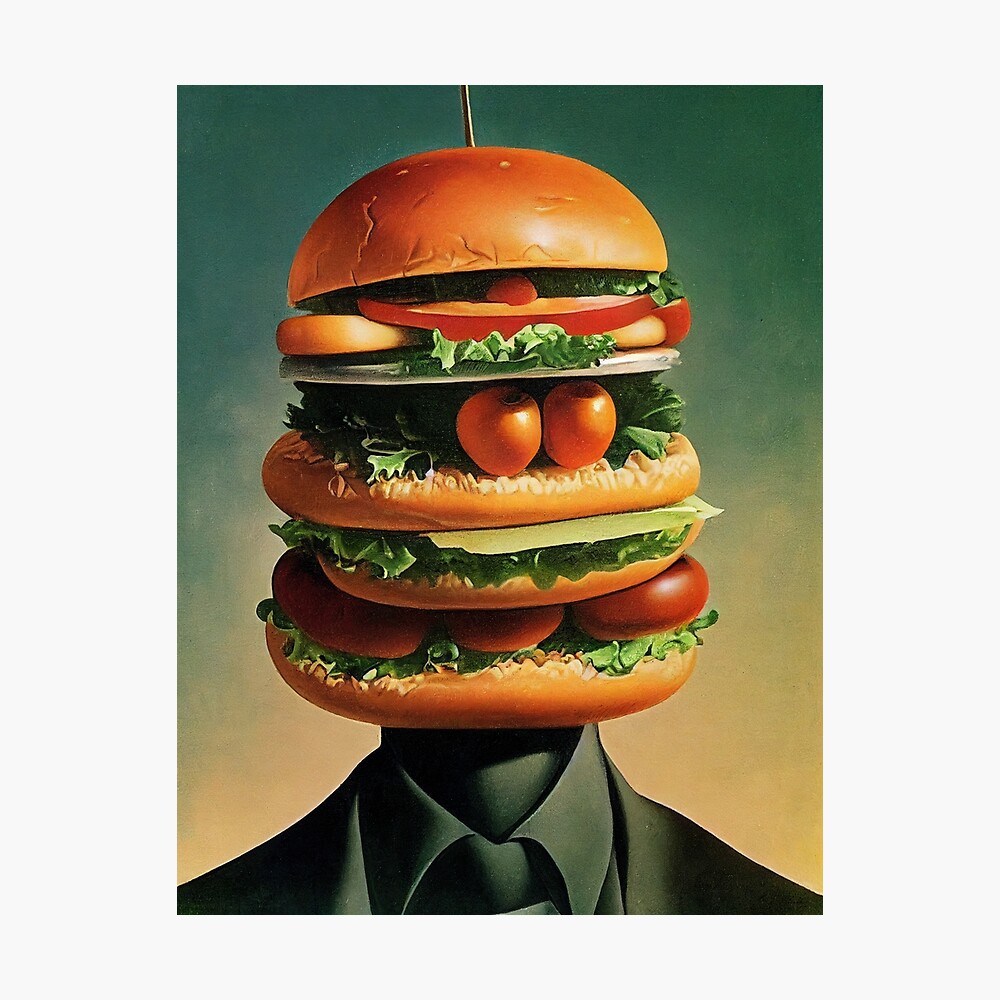This is a highly detailed digital art painting of a man in a business suit whose head has been replaced with a multi-layered, colorful burger. The man is wearing a dark-green suit with a dress shirt visible under the jacket, though it appears to have a stony texture. The burger head is vibrant, with orange buns and layers of lettuce, sliced and squished tomatoes, and multiple buns like a Big Mac, but notably absent of any meat, resembling a vegetable burger. The background is a gradient from dark green at the top to a creamy yellowish hue at the bottom. The rectangular image is framed with a thick, light-gray border.